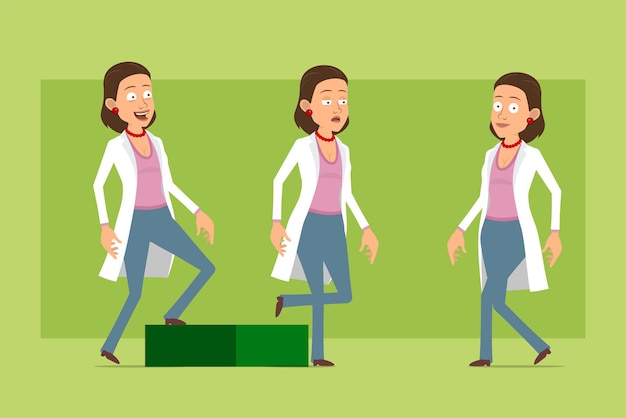The illustration features a cartoon depiction of a woman in three distinct stages of movement, highlighting different expressions and states of activity. The woman, characterized by her brown hair, dons a white lab coat over a pink (or possibly lilac) shirt, complemented by blue pants and brown shoes. She accessorizes with a red necklace and red earrings. 

In the scene on the far left, she is jovially stepping up onto a green box, beaming with a smile, and has a somewhat surprised look. The middle image depicts her stepping down from the box, appearing fatigued. In the final scene on the far right, she is walking towards the left with a normal, attentive expression. The background consists of varying shades of green, with lighter green boxes filling the space. This composition perhaps symbolizes different hours of the day or a cycle of activities and emotions experienced by the woman.